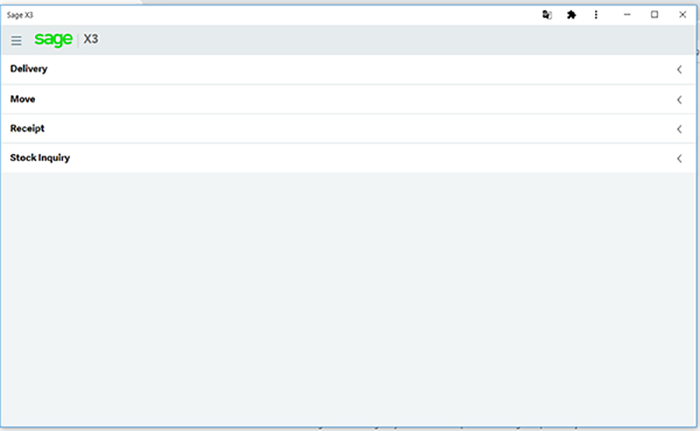A detailed screenshot from Sage X3 is captured in a horizontally rectangular frame. At the very top, a narrow white banner runs across the image, displaying the text "Sage X3" in the upper left corner. On the upper right, several icons are visible: one unclear icon, an extensions icon, and a vertical three-dot menu icon, followed by icons for minimize, maximize, and close functions.

Below this, a narrow gray banner shows a three-horizontal-line menu icon, "Sage" written in green, and "X3" in black. Directly beneath this banner, the main content area features four line items on a white background, labeled "Delivery," "Move," "Receipt," and "Stock Inquiry."

The remainder of the screenshot is a light gray background, devoid of additional text or elements. The entire image frame is delicately outlined with a very thin light blue border.